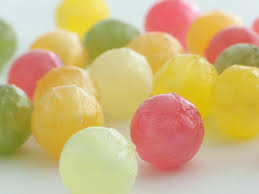The image is a digital photograph depicting an assortment of colorful round candies placed on a white table. The candies, possibly reminiscent of boba pearls, are arranged in a small cluster and are sharply focused while the background remains blurred. The assortment includes candies in a variety of colors: five pink, eight yellow, four green, and two white. Additionally, a light green and dark green presence can be observed, and some viewers mentioned red or orange, which may be perceptual variations. The vibrant candies contrast distinctly against the white, flat surface they rest on, creating a visually appealing and colorful arrangement.